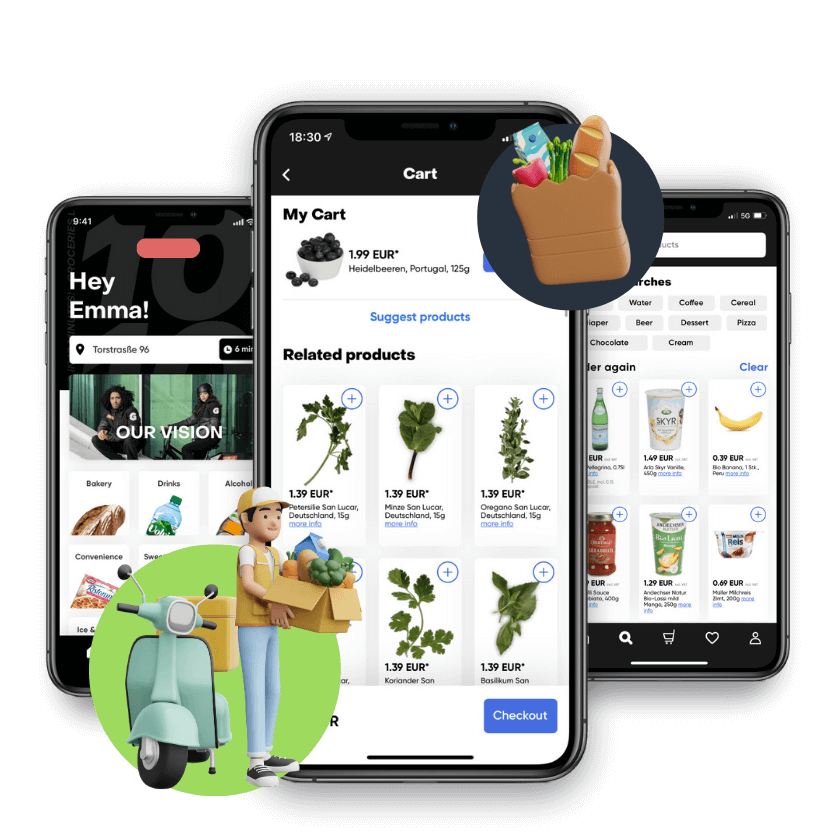The image appears to be of a European grocery store's delivery app interface. At the center of the screen, a banner says "Hey Emma, we got three phones here." Each phone screen displays different sections of the app.

The first phone screen showcases the app’s delivery service, with an icon of a scooter delivering groceries at the bottom. Above it, there are icons for bread and a grocery bag, both nested within green and black circular icons. The brown grocery bag icon contains various groceries while the green icon features a scooter with a delivery person carrying a box of groceries. 

Next to that, there’s a section titled "Our Vision" with subsections like "Bakery," "Drinks," "Alcohol," and "Convenience." Unfortunately, some of the text is obscured by the scooter icon. 

The second phone screen displays a category for spices, likely various herbs, and lists their prices and related products. One tag reads "125 grams" and "€1.99," possibly in reference to items like Hello berries from Portugal.

On the third phone screen, there are images of yogurt products, bananas, and other dairy items, each accompanied by their respective prices. 

The overall impression is that of a comprehensive delivery app designed to meet various grocery needs, indicative of a European market.